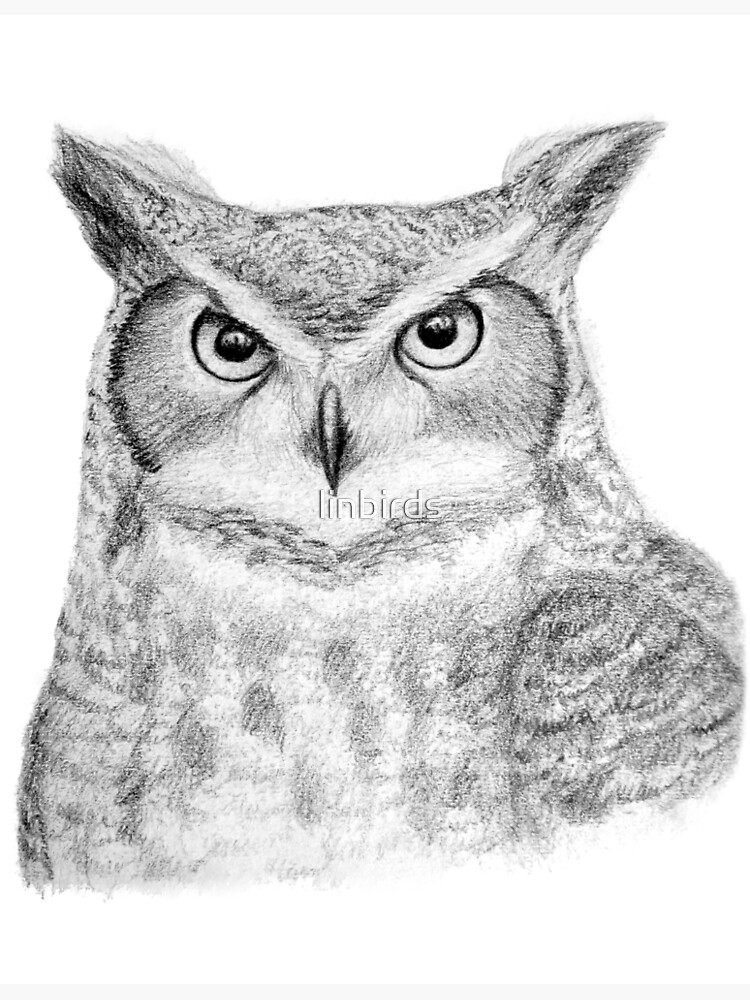This is a highly detailed charcoal sketch of a horned owl rendered in black and white. The owl is facing directly at the viewer with an intense gaze, capturing its head down to mid-chest. The drawing showcases meticulous detail, with each feather individually illustrated, creating a lifelike appearance accented by subtle smudging to emphasize the owl's wispy feathers. The softened lines and visible pencil strokes add texture, making the feathers and facial features, such as the eyes and beak, strikingly realistic. The background is a stark white, highlighting the owl's detailed form. In the center of the image, there is a faint watermark that reads "Linbirds." This artwork, with its refined detail and realistic touch, exemplifies the skill of a very talented artist.